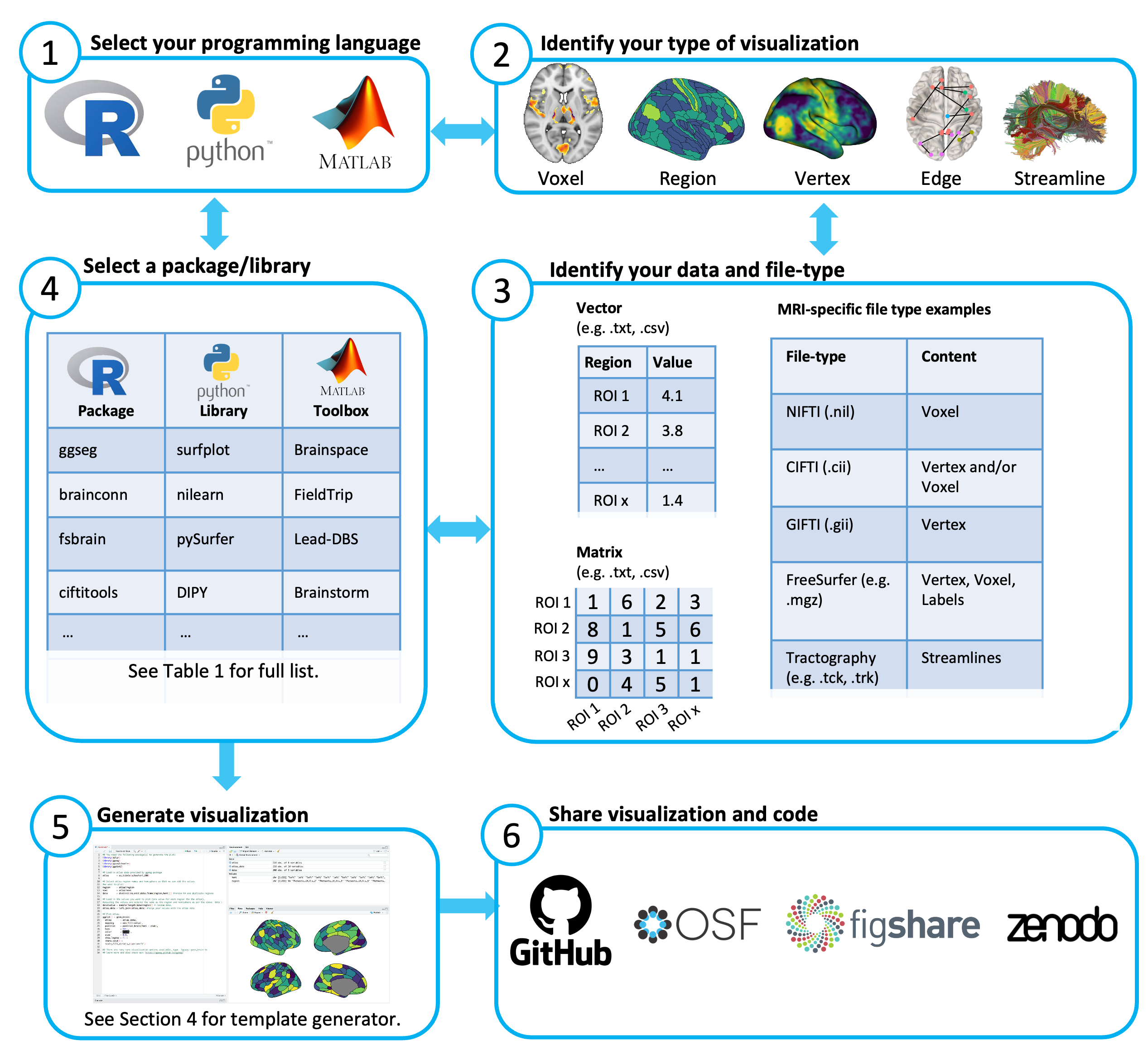The image is an instructional flowchart detailing a six-step process for generating and sharing visualizations from programming languages. At the top left, Box 1 is labeled "Select Your Programming Language," featuring logos for R (a blue 'R' with a gray circle), Python (blue and yellow Python logo), and MATLAB (MATLAB logo). Box 2 instructs to "Identify Your Type of Visualization," listing options such as voxel, region, vertex, edge, and streamline, illustrated with images resembling brain structures. Below, Box 3 asks to "Identify Your Data and File Type," providing examples like text or CSV, matrix, and MRI-specific file types. Box 4, "Select Package and Library," displays logos for R, Python, and MATLAB. Box 5 guides users to "Generate Visualization," showing a screenshot of code and visual outputs, with a note to see section 4 for a template generator. The final step, Box 6, advises to "Share Visualization and Code," mentioning platforms like GitHub, OSF, Figshare, and Sonata. This detailed and technical flowchart is ideal for educational settings, such as college classrooms or textbooks, providing a clear and systematic approach to data visualization.